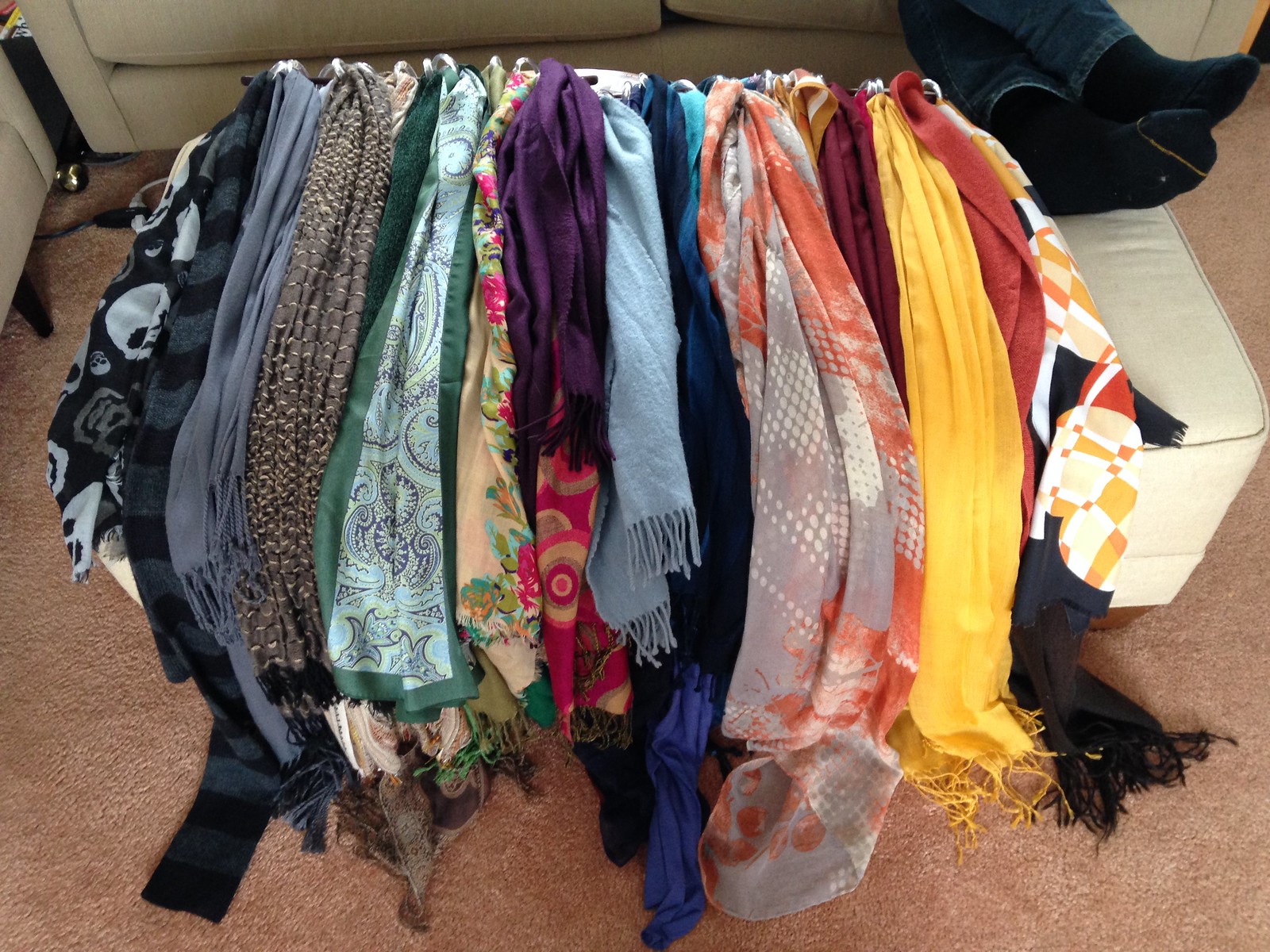The image showcases a cozy living room scene centered around a collection of beautiful neck scarves. Spread out on a cream-colored footrest in front of a light tan-colored sofa, the scarves create a vibrant display of colors and patterns against a beige carpet. Among the assortment, there’s a striking black scarf adorned with silvery skulls, a solid blue scarf, a purple one, and another sporting green and pink flowers. The scarves vary in length and include designs ranging from solid colors to intricate patterns, including one that looks Indian-inspired and another featuring a dark gray line pattern. Resting casually on the footrest, a pair of legs clothed in jeans and black socks adds a relaxed, homey touch to the scene. The beige sofa, partly visible in the background, along with the soft peach-toned carpet, frames this inviting and colorful display.